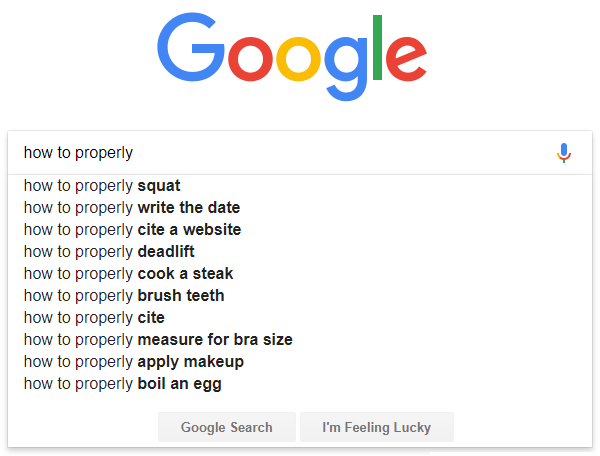The image is a screenshot of a Google search where the user has started typing "how to properly." The Google logo, with its characteristic colors, is prominently displayed at the top. The logo consists of a capital 'G' in blue, a lowercase 'o' in red, another lowercase 'o' in yellow, a lowercase 'g' in blue, a lowercase 'l' in green, and a lowercase 'e' in red. In the search bar, the phrase "how to properly" is partially typed, followed by a blue microphone icon indicating voice search.

Below the search bar, Google’s autocomplete suggestions are listed. Each suggestion shows the phrase "how to properly" followed by specific actions, with the action words bolded. The suggestions are as follows: 
1. "how to properly squat" (with "squat" bolded)
2. "how to properly rate the date" (with "rate the date" bolded)
3. "how to properly cite a website" (with "cite a website" bolded)
4. "how to properly deadlift" (with "deadlift" bolded)
5. "how to properly cook a steak" (with "cook a steak" bolded)
6. "how to properly brush teeth" (with "brush teeth" bolded)
7. "how to properly cite" (with "cite" bolded)
8. "how to properly measure for bra size" (with "measure for bra size" bolded)
9. "how to properly apply makeup" (with "apply makeup" bolded)
10. "how to properly boil an egg" (with "boil an egg" bolded)

At the bottom of the screen, the familiar "Google Search" and "I'm Feeling Lucky" buttons are visible. This screenshot captures a moment of curiosity as the user seeks guidance on various tasks.